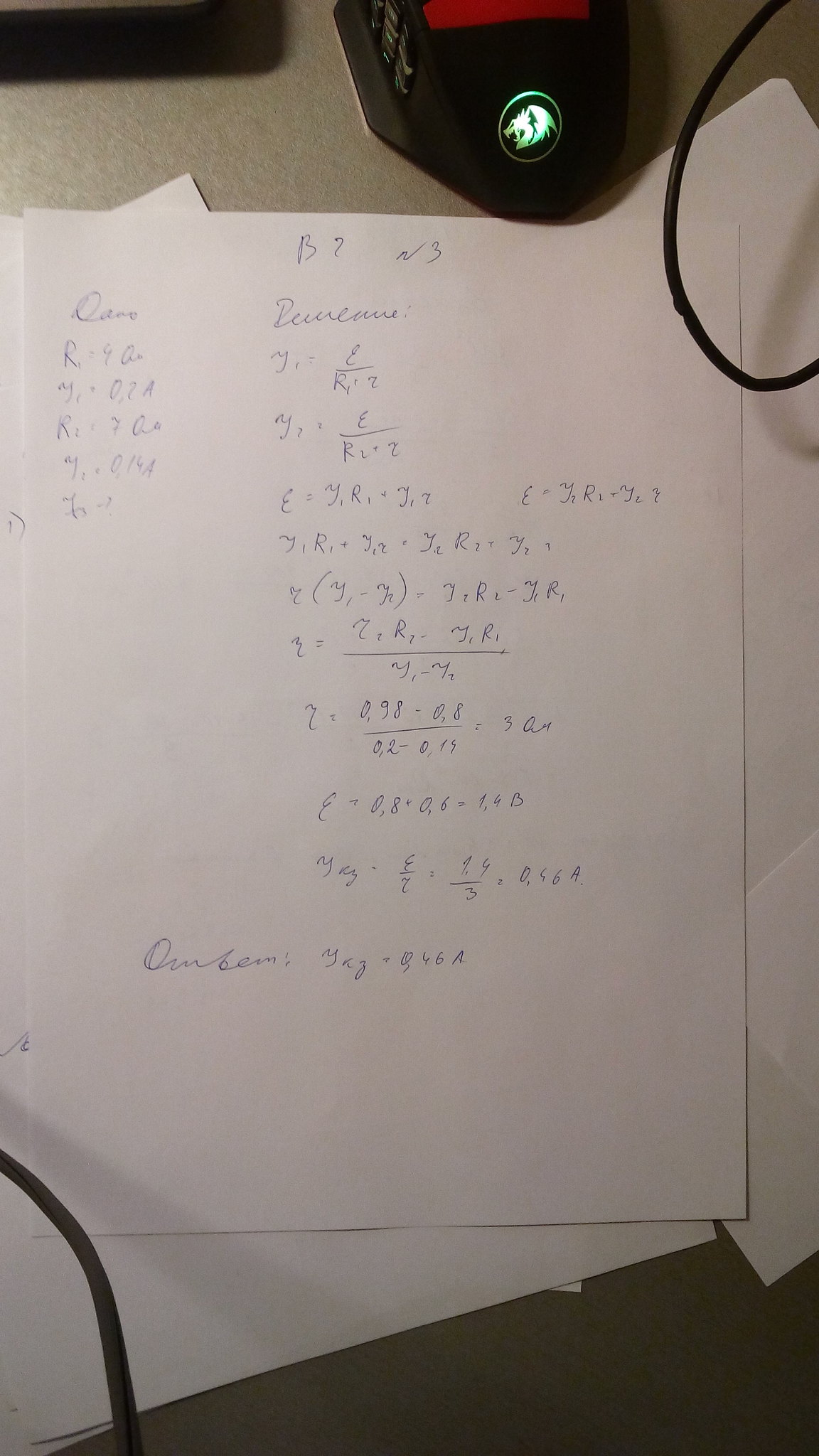The image presents a detailed overview of a piece of paper adorned with handwriting in blue pen. The script is cursive, and the content includes a mix of letters and intricate numerical calculations. The writing, however, is somewhat challenging to discern due to its small size and the image's clarity. Beneath the primary piece of paper lie two additional sheets of white paper—one angled to the left and the other positioned slightly lower and side by side. At the very top of the image, a portion of a computer mouse and a cord can be seen in the upper right. Another cord is visible in the bottom left corner of the image. Just above the center near the bottom, a tiny corner of yet another piece of paper peeks out from under the other sheets. In the upper left, a shadow is cast, revealing the papers rest on a light gray or light brown surface.